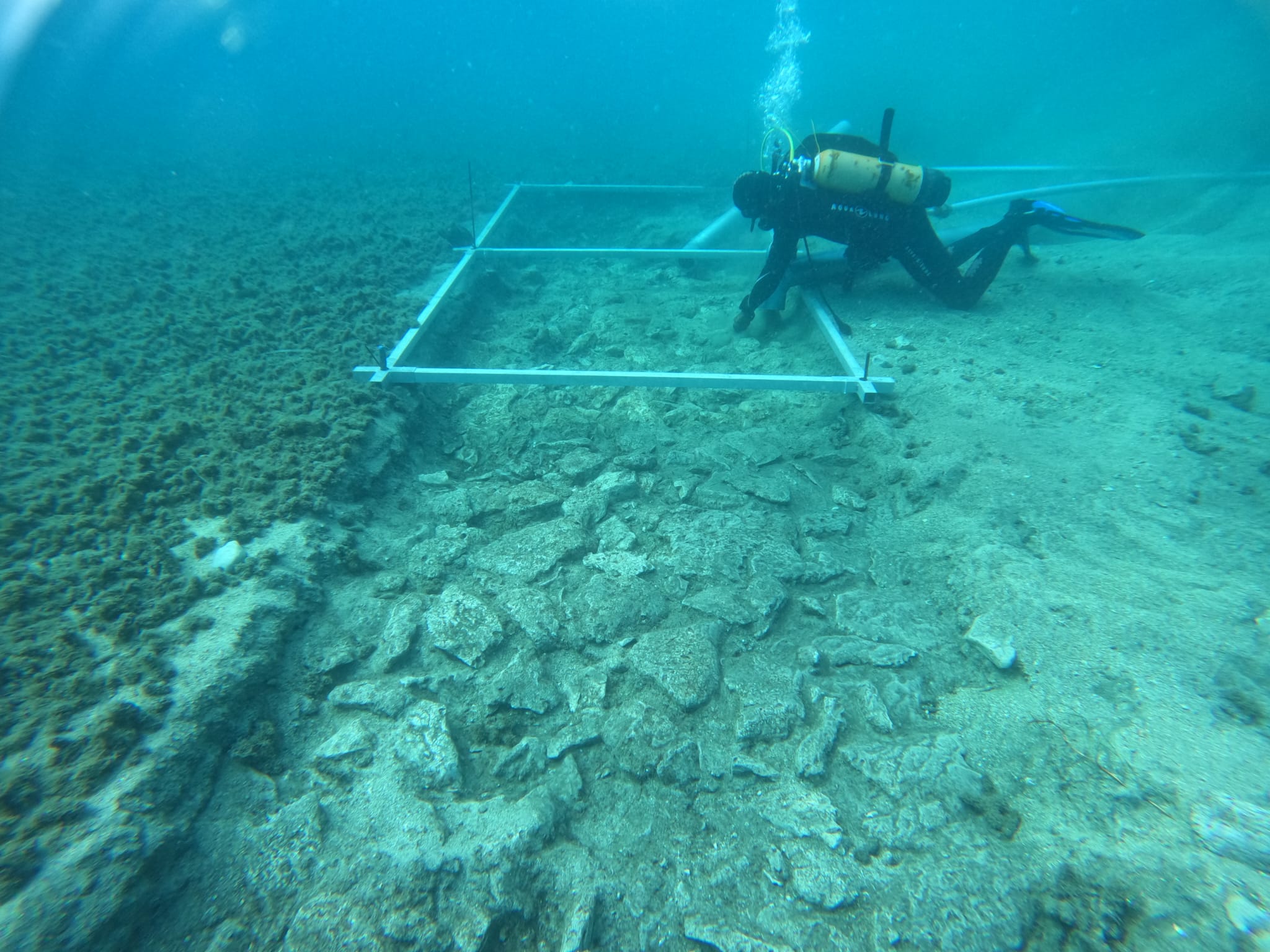The image showcases an underwater diver, fully equipped with a scuba suit, flippers, and an oxygen tank, releasing bubbles as he works. The background water is a deep, hazy blue, with streaks of sunlight filtering down from the upper left, creating a softly illuminated ambiance. The diver is actively assembling a metal structure consisting of white or metallic squares fastened together with metal rods. He is currently working on the second square, while the first is positioned to his right, further back in the image from the viewer's perspective. This metal frame appears to be affixed to a squared-off area of rock, suggesting ongoing construction or repair. The underwater scene also hints at moss or plant life on the left side, adding to the aquatic environment's authenticity. Despite the foggy depth, the diver seems to be near the surface, focused intently on his underwater task.